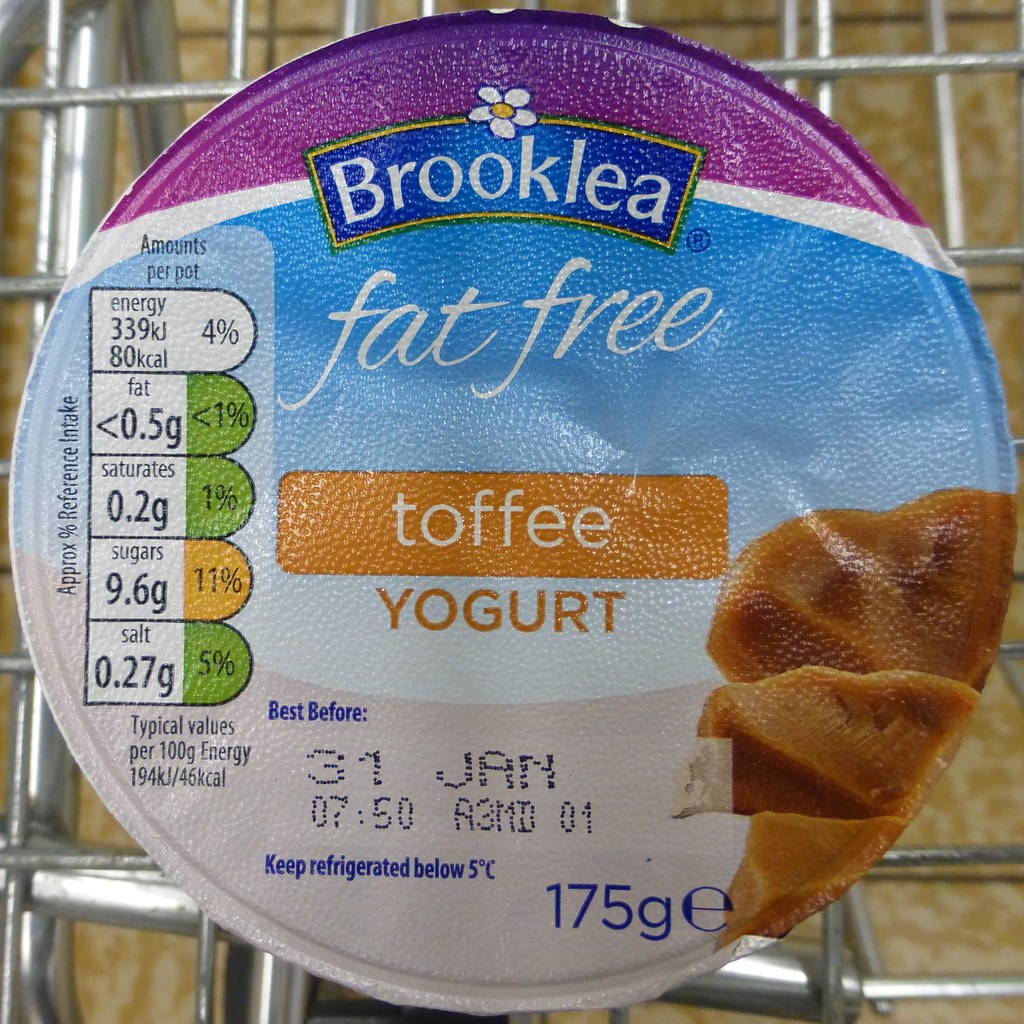The photograph features a close-up of the top label of a yogurt container resting on what appears to be a silver shopping cart, with glimpses of the yellow and white tiled floor in the background. The lid design prominently displays the brand name “Brooklea” in white letters, outlined in blue, set against a purple background. A white daisy with a yellow center serves as a decorative element above the brand name.

Immediately below, the label indicates "fat-free" in white letters on a blue background. Towards the center, an orange tab inscribed with “toffee” in white letters highlights the flavor of the yogurt, which is further denoted as "yogurt" in orange letters on a white background. Surrounding these key text elements are important nutritional details including energy, fats, saturates, sugars, and salt content, each listed with precise measurements in grams and percentages per serving, all in black letters on a white background.

Additional information includes the expiration date, "Best before January 31," and storage instructions, "Keep refrigerated below 5°C," printed in blue letters on a white background. The label also lists the net weight of the product as 175 grams. The detailed and colorful design elements ensure clarity and provide comprehensive information about the yogurt.